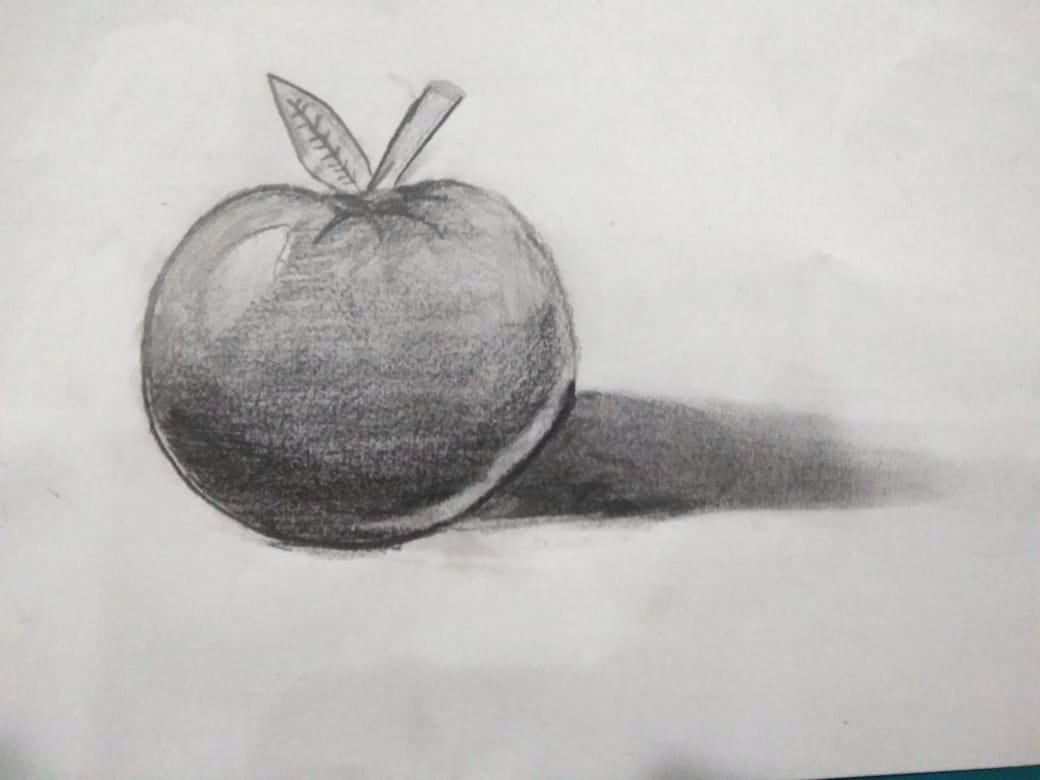This detailed black and white photograph captures a pencil sketch of an apple, set against a slightly wrinkled white paper that reveals the edge of a table surface in the corner. The apple, accurately identified by its short stem and small leaf, is rendered with meticulously shaded textures. The shading ranges from light gray to deep black, accentuating the apple's round, spherical form and providing a rich sense of dimensionality. A distinct eye-shaped highlight on the upper side of the apple suggests a light source coming from the left. Below, the apple casts a shadow that is darker near its base and gradually lightens as it extends outward, mirroring the direction of the light.